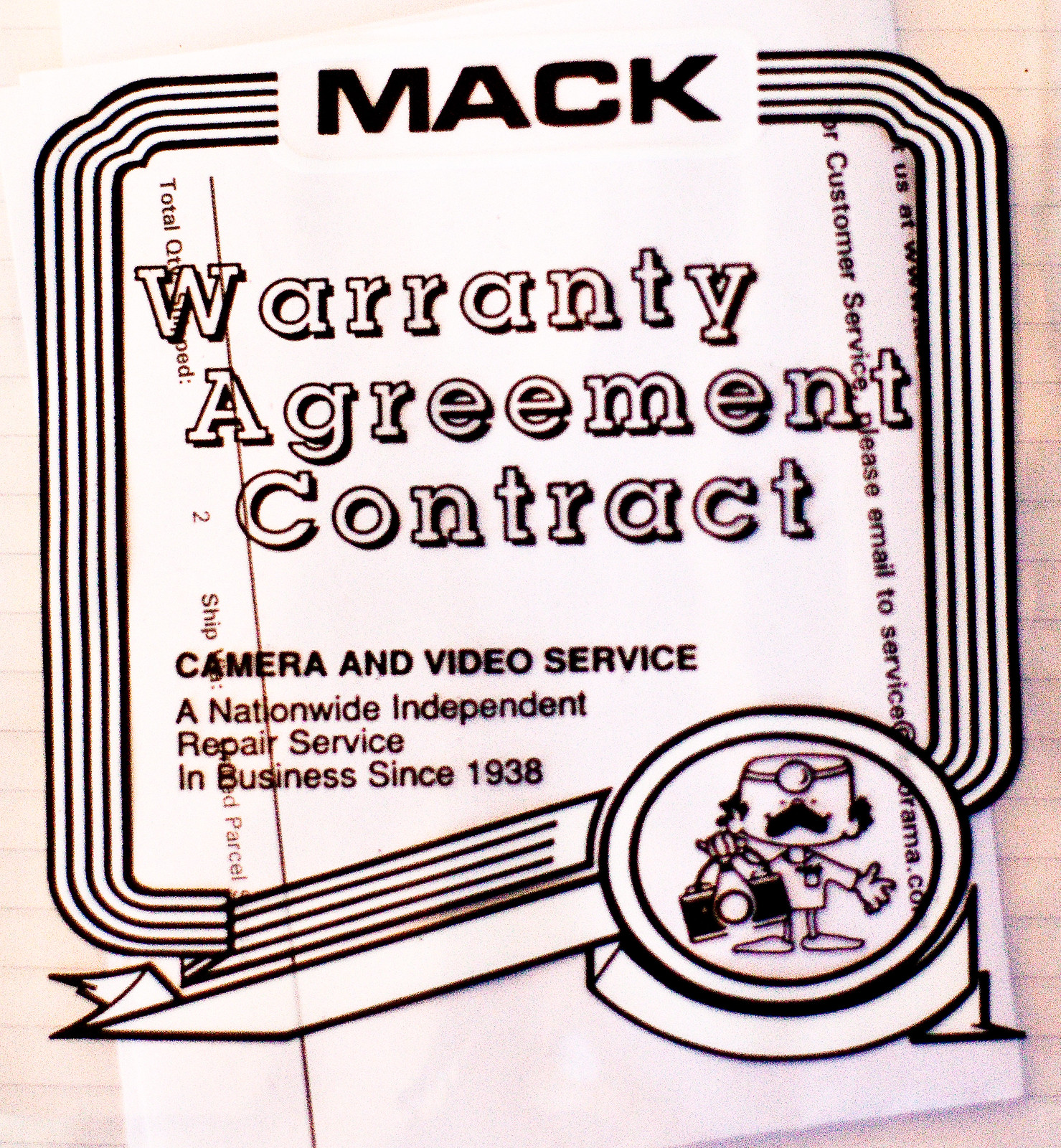This image appears to be a poster or advertisement for a warranty agreement contract by a company called MAC, which specializes in camera and video service. MAC has been a nationwide independent repair service since 1938. Prominently featured at the top of the image are the words "MAC Warranty Agreement Contract, Camera and Video Service," emphasizing the company's long history and nationwide presence. The image predominantly uses black, white, and tan colors. The paper or label takes up the entirety of the image, suggesting it's a formal document. In the lower right corner, there's a cartoon icon of a mustached man, depicted as a doctor, holding a camera. This character is surrounded by a ribbon in one description and is printed on clear plastic in another, overlaying the agreement underneath. The setting suggests this is the kind of contract you would receive from a camera repair company, with clear visual branding and detailed presentation emphasizing professionalism and longevity of the service.